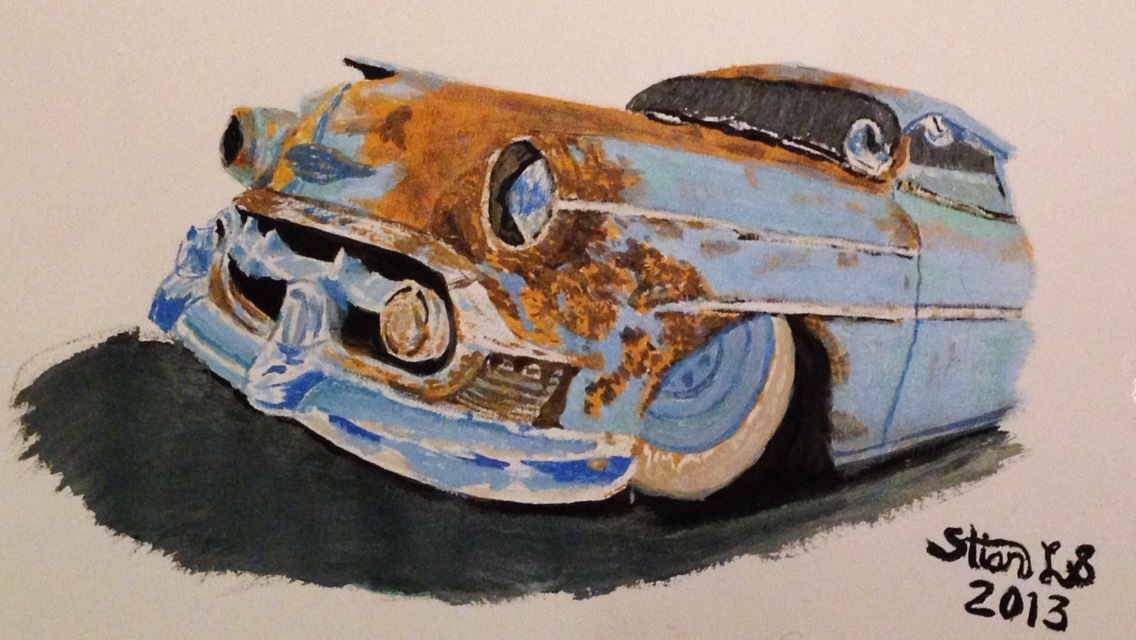This watercolor painting displays the front half of an old, rusted car, prominently placed in the center of a tan rectangular canvas. The vehicle, originally a powder blue or Carolina blue, is depicted traveling from left to right, with its headlights on the right side. Its dilapidated exterior is marred by extensive rust around the headlight areas, the hood, the front windshield, the fender, the roof, and notably over the wheel. The headlight on the left side is notably missing. The car’s tires feature thick white-walled rims that share the same powder blue hue. Beneath the vehicle, a black shadow adds depth to the scene. Detailing a fine blend of artistry and decay, the piece captures the essence of automotive aging with vivid rust spots in shades of brown. In the bottom right corner, the artist’s signature, reading "STIANLB 2013," is inscribed in black paint.